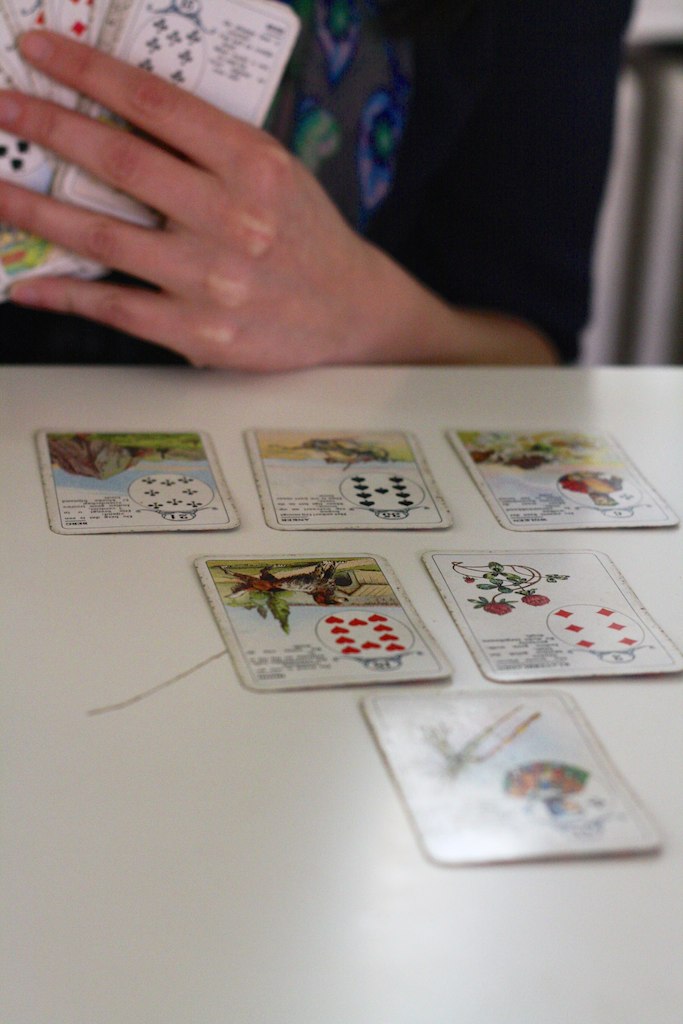A white table serves as the stage for six uniquely illustrated cards arranged in an upside-down pyramid. In the background, a Caucasian hand, clad in a vibrant black, blue, and green shirt, fans out additional cards. These cards aren't typical playing cards like the familiar Bicycle brand but feature distinctive images. The central two cards display intricate designs: the left card boasts a circle of ten hearts, while the right showcases six diamonds arranged similarly. On the bottom row, the card on the far right is identifiable as the Eight of Clubs due to the circular arrangement of eight club symbols, and the center card is the Nine of Spades, marked by nine spades in a circle. The images on the cards are intricate and appear upside-down, lacking any textual identifiers such as "King of Spades" or "Six of Diamonds."